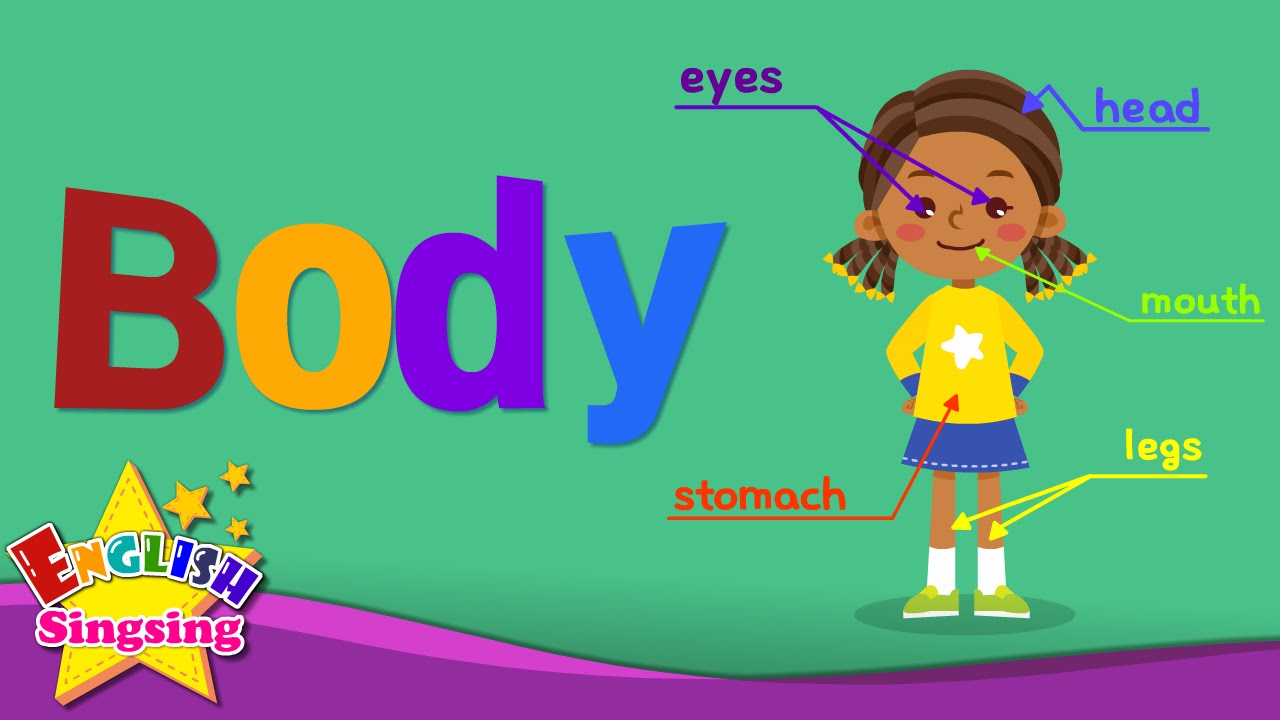This vibrant, colorful children's illustration features a cheerful educational theme. The image is approximately twice as wide as it is tall, with a predominantly green background transitioning to a purple wave design at the bottom. On the left side, the prominent word "body" is written in large, colorful letters: a red 'B', an orange 'O', a purple 'D', and a blue 'Y'. 

In the bottom left-hand corner, a yellow star contains the text "English Sing Sing" in a variety of colors, with "English" being multicolored and "Sing Sing" in pink, surrounded by a few smaller stars. 

Dominating the right side is a young black girl with pigtails, dressed in a cheerful outfit resembling a cheerleader's uniform: a yellow long-sleeve bodice with a blue skirt, white socks, and lime green shoes. She stands with a confident, smiling posture, hands on her hips. Various parts of her body are labeled with colorful arrows: "eyes" in purple, "head" in blue, "mouth" in lime green, "legs" in yellow, and "stomach" in orange. The playful and instructional design makes it a delightful learning tool for children.